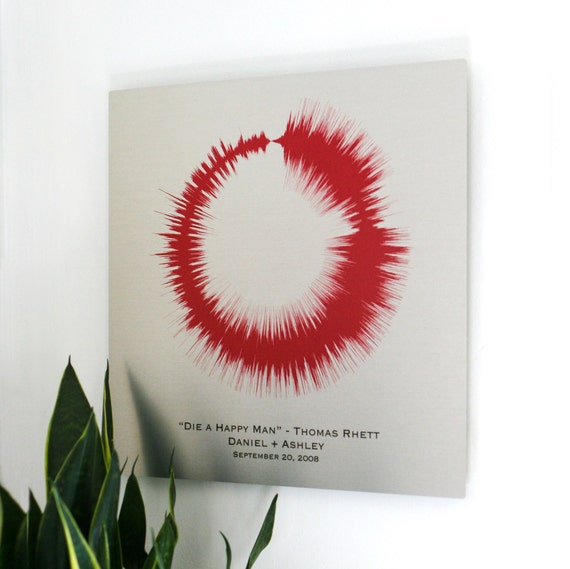The image depicts a square canvas hanging on a large white wall within an indoor setting, possibly a home or museum. The canvas features a light gray background with a prominent red circle at its center. The circle has an irregular, jagged edge, as if the wet paint was crisscrossed with a string, creating a striking and textured appearance. Beneath the circle, in bold black text, there is an inspirational quote that reads, "Die a Happy Man," attributed to Thomas Rhett. Below the quote, the names "Daniel + Ashley" are inscribed, followed by the date "September 20, 2008." In the lower left corner of the scene, there is a house plant with dark green leaves and yellow accents, adding a touch of natural contrast to the artistic setting.